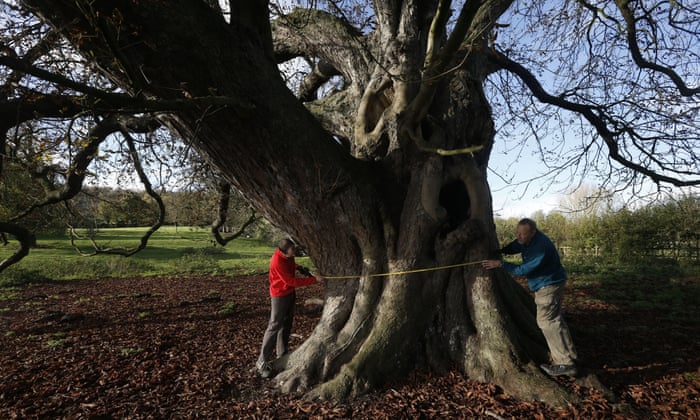The photograph, rectangular in shape with its longer sides at the top and bottom, captures a detailed scene of two men measuring an enormous, leafless tree using a yellow measuring tape. At the center of the image stands the imposing tree, about five people thick in diameter, with its sprawling, curved branches suggesting an ancient presence. On the left side of the tree, a man dressed in gray pants, white shoes, and a long sleeve red shirt holds one end of the measuring tape. On the right, another man, clad in tan cargo pants, black shoes, and a long sleeve blue shirt, grips the other end. The ground around the tree is covered with mulch, creating a noticeable circular base that extends approximately 30 to 40 feet in diameter. In the background, a lush green field dotted with smaller, leafy trees stretches out, set against a bright blue sky, indicating an early springtime setting.